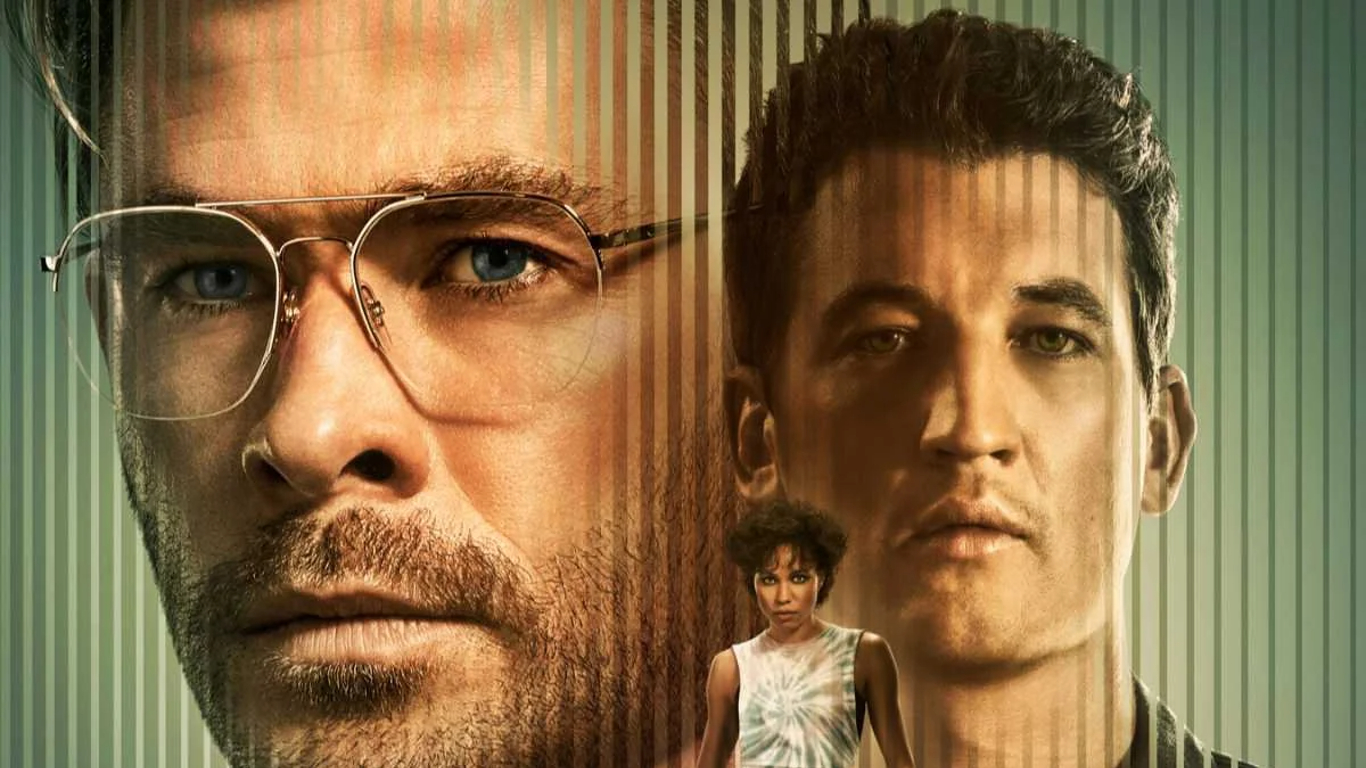The image features a close-up of a man's face prominently on the left side. He has blonde hair, blue eyes, and a light brown goatee and mustache. He is wearing silver rimmed glasses that resemble those famously worn by Jeffrey Dahmer. His face occupies a large portion of the image, emphasizing his broad nostrils and light stubble, suggesting he hasn't shaved in a couple of days. To the right, there's a smaller image of a younger man with dark brown, thick, curly hair and green eyes. He is clean-shaven with a dimpled chin, and his facial expression is directed straight at the camera, reminiscent of Elvis. Between these two men is a significantly smaller image of a black woman, visible from her head to her waist, positioned in front of their faces. She has short, curly black hair that’s high and a hint of muscular arms. She is wearing a sleeveless, tie-dye swirl shirt. The entire photograph has a transparent overlay of light green stripes that fade out completely in front of the faces, giving the image a distinctive textured background with darker green and dark green stripes, almost resembling a movie poster or an artistic painting.